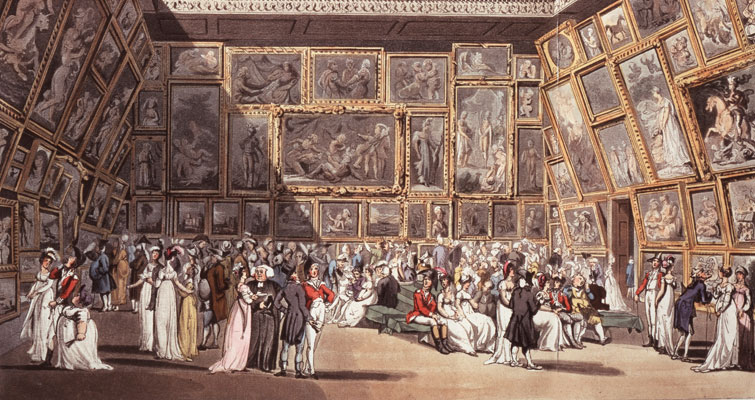This image depicts a grand, historical interior, possibly of a Victorian-era museum or gallery, adorned with intricate scrollwork on the ceiling. The walls, covered with an array of drawings varying in shapes and sizes, are framed with ornate gold and gilded frames. These framed artworks span from the floor to the ceiling across the left, back, and right walls. The drawings prominently feature people, and their subjects are rendered in a black and white style at the top.

On the ground level, the floor presents a grayish tone, and though faint, numerous people can be seen occupying the expansive space. The visitors, dressed in period attire, contribute to the historical ambiance. The attire includes elegant white gowns, red gowns, and black gowns for the women, while the men are clad in long black coats, white pants, and tall boots, with several donning powdered wigs.

In the foreground, three women stand facing the pictures on the left wall—two in white gowns and one in a striking red gown. Near the center left, a small group draws attention: a woman in a white gown facing right, beside a man with white hair in a black gown who is looking toward her, followed by a man with a black jacket and white pants, and behind him, a woman in white pants, a red shirt, and a black hat facing the camera.

Throughout the scene, the crowd reflects a blend of French and possibly English Victorian styles, with the presence of soldiers reminiscent of historical figures like Bonaparte. The rich details and the collective attire create an immersive experience, suggesting a moment lifted from history, capturing the essence of an old, esteemed museum filled with people appreciating the artistry surrounding them.